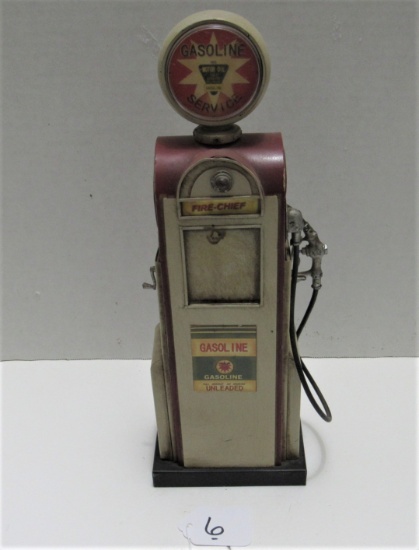This image features a detailed miniature model of an old-school gas pump, likely intended for use with a model train set or similar display. The gas pump is predominantly a dark burgundy-red color, with a mix of silver or gray accents. It stands on a white surface against a gray background, resembling a vignette on a white table with a gray wall behind it. The model is characterized by its rectangular body, rounded top, and circular signage above.

At the very top, the circular sign is maroon with a white star in the center and includes black text that reads "Gasoline Service." The rounded top of the gas pump continues the maroon hue, transitioning to a white rectangular body with the words "Fire Chief" prominently displayed. Further down, another label reads "Gasoline" in red text, accompanied by additional writing below it, which is harder to decipher. A silver spout, presumably the pump handle, is attached to the right side, and there appears to be a crank on the left side of the model. The entire gas pump is mounted on a black pedestal, and a small piece of paper labeled with the number 6 is placed beneath the model.